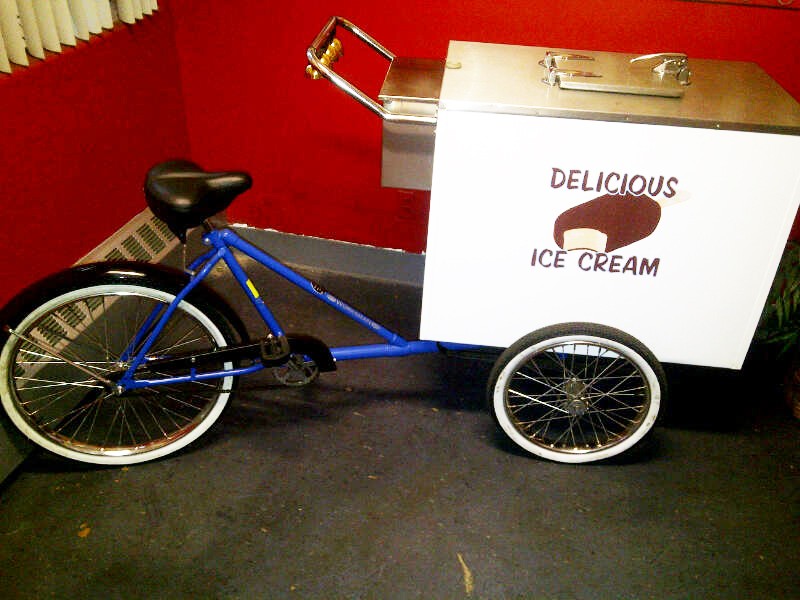This image shows a long, blue bicycle with a black seat, standing inside a room with cherry red walls, possibly featuring curtain blinds and a wall heater in the background. Attached to the front of the bicycle is a white chest freezer, designed to look like a classic ice cream cart. The freezer features a silver top with an opening for accessing the ice cream stored inside, and prominently displays the text "Delicious Ice Cream" along with an image of a bitten ice cream bar. The handlebars of the bike extend from this freezer box, indicating that it is used by someone who rides the bike to sell ice cream.